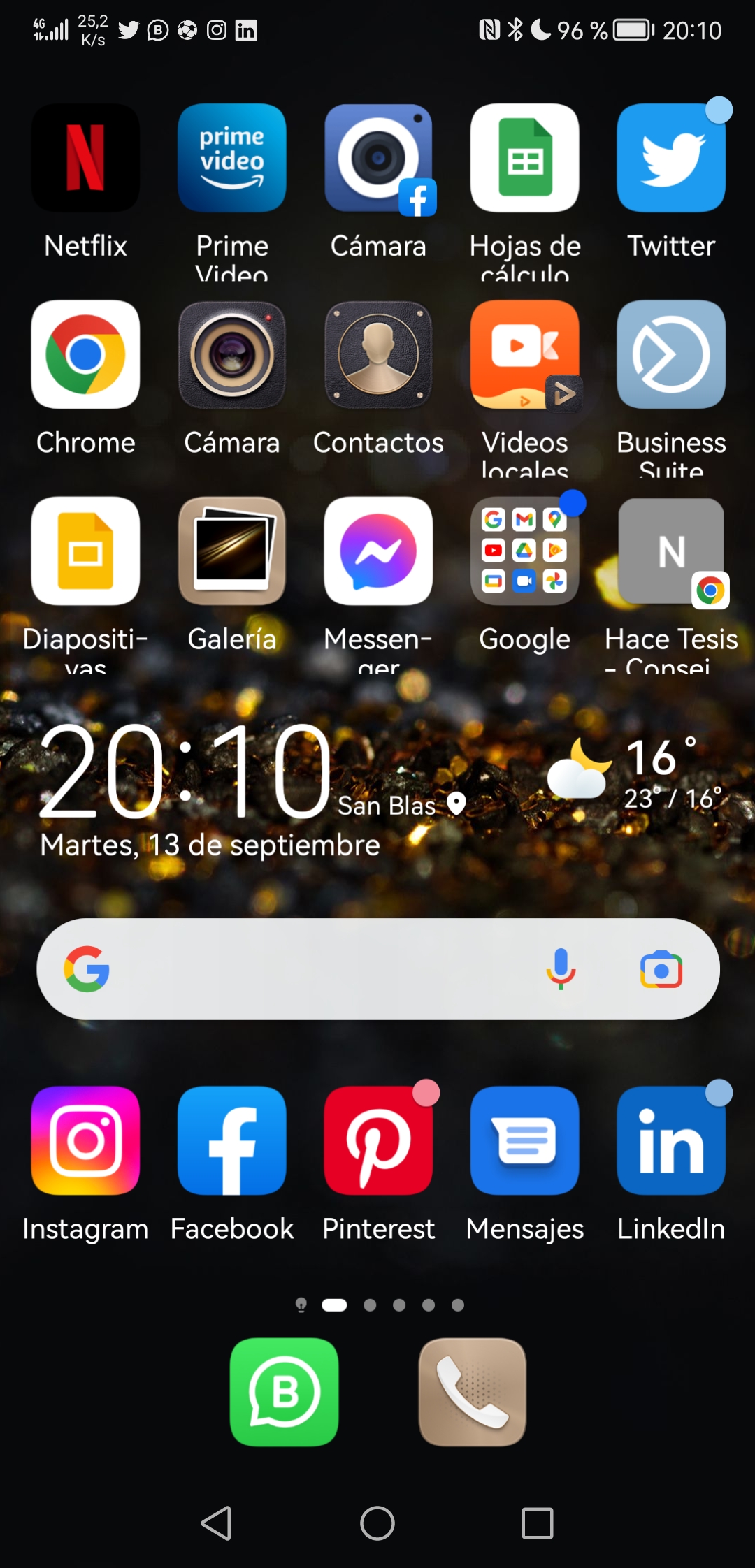This image is a screenshot taken from a smartphone, showcasing its home screen. The status bar at the top brims with various symbols: the time displayed on the right as 20:10, a fully charged battery icon at 96%, a crescent moon symbol indicating Do Not Disturb mode, a Bluetooth symbol, and an NFC (Near Field Communication) icon.

The background of the screenshot is predominantly black, featuring a central wallpaper that resembles outdoor gravel with glimmering gold sparkles scattered throughout. The textures range from black to dark grey with bronze tones, presenting an appearance that could be interpreted as either gravel or glittering gemstones. The wallpaper is slightly out of focus, making it challenging to discern as it's partially obscured by the screen's widgets and icons.

A clock widget positioned on the center-left displays the time as 20:10 in large white text. Below it, the date is shown in Spanish, reading "MARTES, 13 de Septiembre," indicating it is Tuesday, the 13th of September. 

Moving to the icons of the apps on the device, located at the top left of the screen, there is a row of applications. These include Netflix, Prime Video, and the Camera app. Notably, the Camera app is labeled in Spanish as "CÁMARA," with an accented 'A'.

The screenshot provides a glimpse into a multilingual smartphone setup with a neatly organized yet intricate home screen layout.